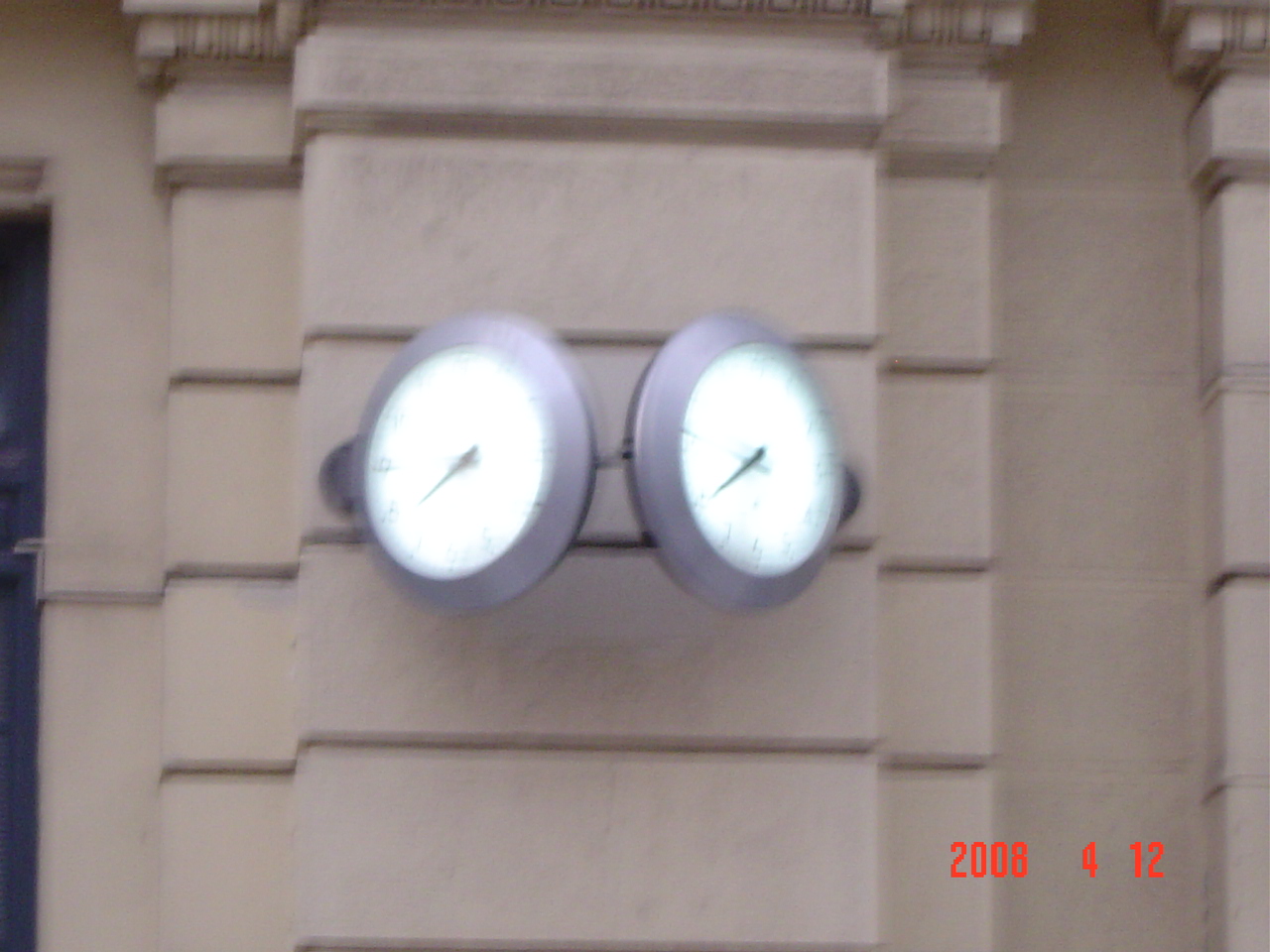This image captures the side of a building adorned with statuesque columns, albeit with some blur. Each column is divided into five discernible sections, and the particular column in the middle prominently displays this structural detail. Affixed to this column are two substantial, almost pewter-colored metal clocks with white faces, which appear to be backlit. Despite the image's blurriness, the clocks' black writing and hands, including the second hands, are faintly visible. For clarity, the image was taken on April 12, 2008, as indicated by a date stamp at the bottom. To the left of the image, a sizable black door adds to the architectural intrigue of the building's exterior.